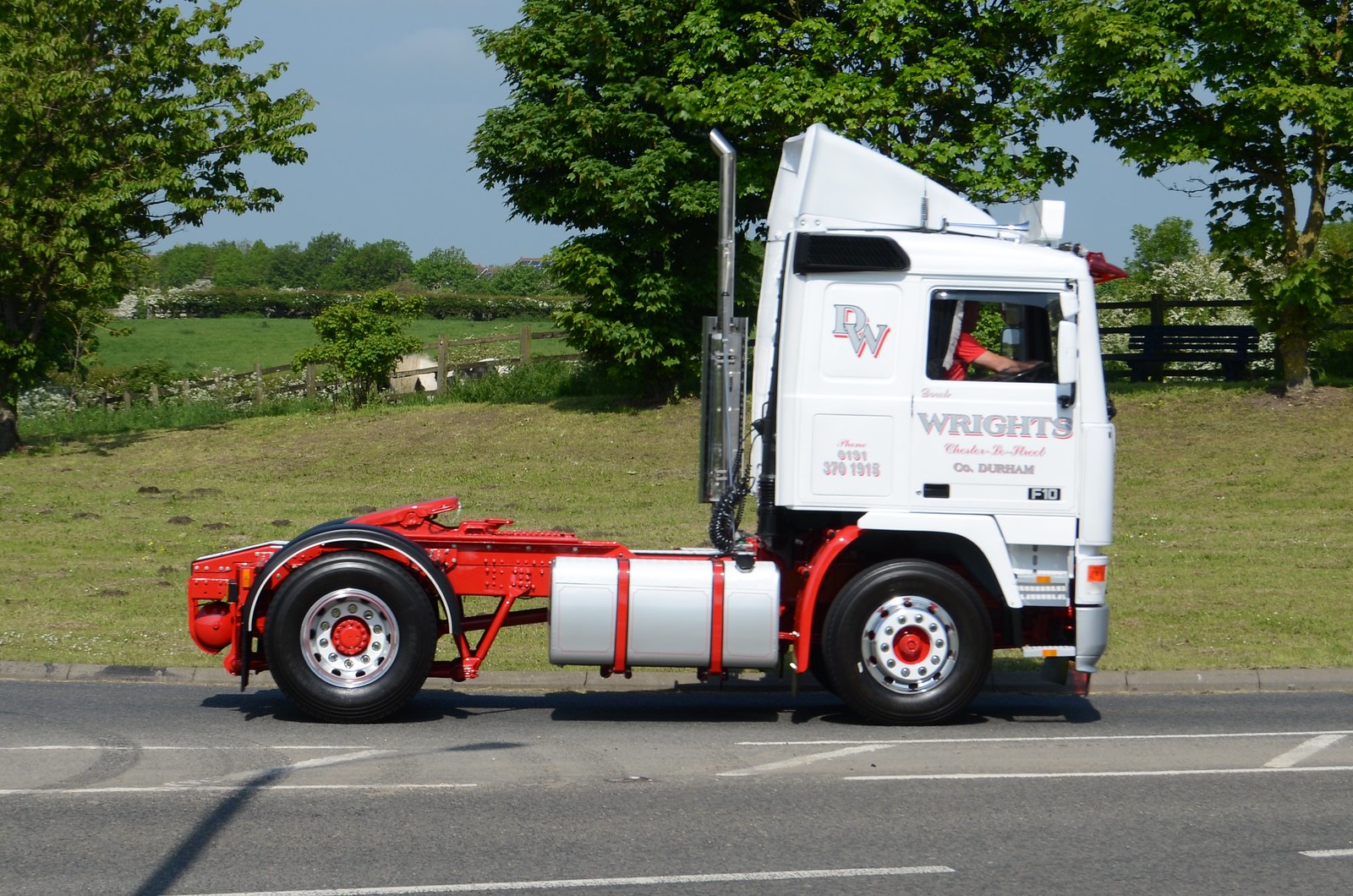The image captures the right-hand side view of a semi-tractor trailer without the trailer, revealing its white, cubic cab with red and gray text. Displayed on the upper left of the cab are the capital letters "DW", and on the side are the words "WRIGHTS" along with various smaller inscriptions, though some text is too small to read clearly. The vehicle features a red chassis, a gray rectangular tank, and shiny chrome exhaust pipes at the rear of the cab. The driver, a white man in a red short-sleeved T-shirt, appears to be driving on the right side, suggesting the location might be in England. The road, gray with white lines, lies in the foreground while the background showcases a picturesque countryside scene with a lush, green meadow, a man-made wooden fence, tall green trees, a scattering of flowers, and a brilliant blue sky.